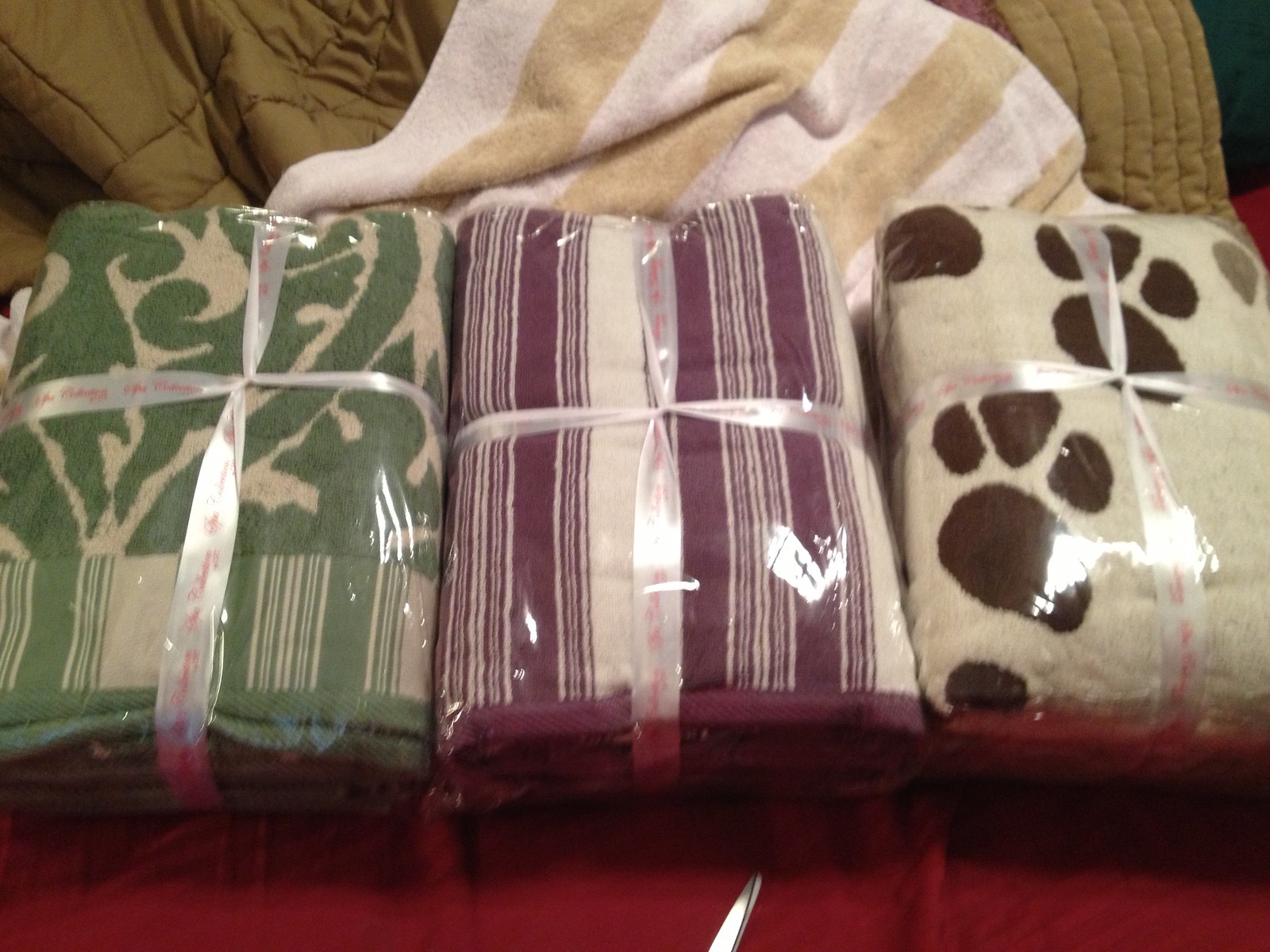The image features three individually wrapped blankets, each designed with unique patterns and presented horizontally across the photograph. From left to right:

1. The left-most blanket is predominantly green with a white pattern overlay. It features thin white stripes centrally bordered by green sections, and is edged with a striped design, adding a textured look. This blanket is encased in clear plastic packaging and adorned with a satin white ribbon featuring pink writing.

2. The middle blanket boasts a pattern of thick burgundy stripes and thinner variations, juxtaposed with larger cream stripes. This vertically striped design is similar in packaging, also wrapped in clear plastic and tied with the same type of satin ribbon.

3. The right blanket has a cream-colored base decorated with large brown paw prints, each print detailed with one large pad and three smaller ones. Like the others, it’s neatly wrapped in plastic and a satin ribbon.

The backdrop appears to be a bed, with additional towels or blankets spread around, contributing to the cozy and organized arrangement.